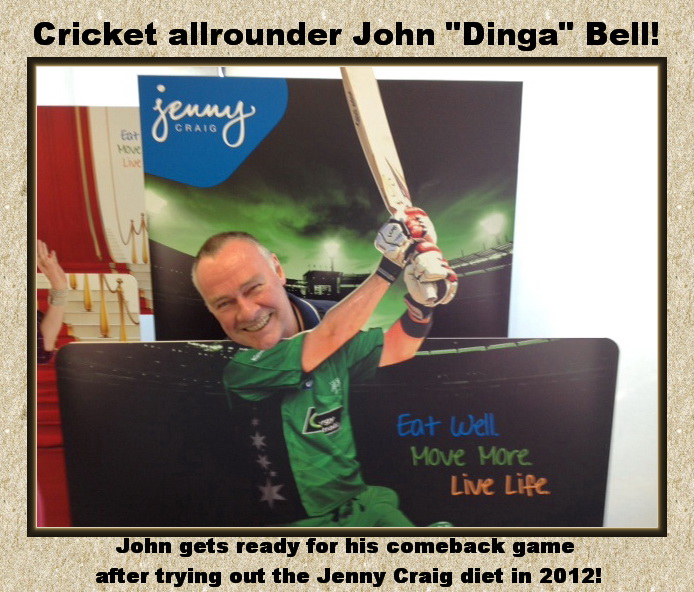This detailed color photograph, framed in brown with a black border, prominently features a cricket player, identified at the top in black letters as "Cricket All-Rounder John 'Dinga' Bell!" John Bell, captured mid-swing with a cricket bat in his gloved hands, wears a green uniform with black stripes and a star on the jersey, matched with green shorts. His complexion is light, with short, black and gray hair receding at the sides.

The background of the image includes a blue sign with white letters reading "Jenny Craig" and a multi-colored motivational message: in blue letters "eat well," in green letters "move more," and in orange letters "live life," all set against what appears to be the sky above a stadium. Below, a black text caption reads: "John gets ready for his comeback game after trying out the Jenny Craig diet in 2012!" The overall scene is brightly lit by natural light, enhancing the clarity and vividness of John's determined and smiling expression as he stands ready for his cricket comeback.